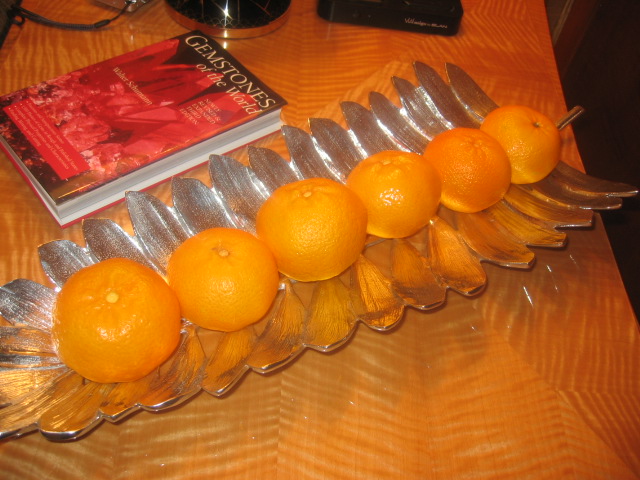The image showcases a meticulously arranged display of six oranges, presented on a slender, silver tray designed to resemble a long, vertical leaf with a slightly curved structure, adorned with leaf-like patterns along its length. The oranges are neatly placed from left to right, varying in size from largest to smallest, and rest atop the tray, which is positioned on a table draped with what appears to be an orange tablecloth. Directly behind this elegant fruit arrangement, a book titled "Gemstones of the World" is prominently visible, featuring a cover with a black background and an array of red gemstones, likely rubies, along with white title text and a distinct red band at the bottom housing additional tiny white text. The image is closely framed, capturing the detailed textures of both the fruits and the metallic leaf tray, while also offering a glimpse of two other indistinguishable black items positioned behind the book.